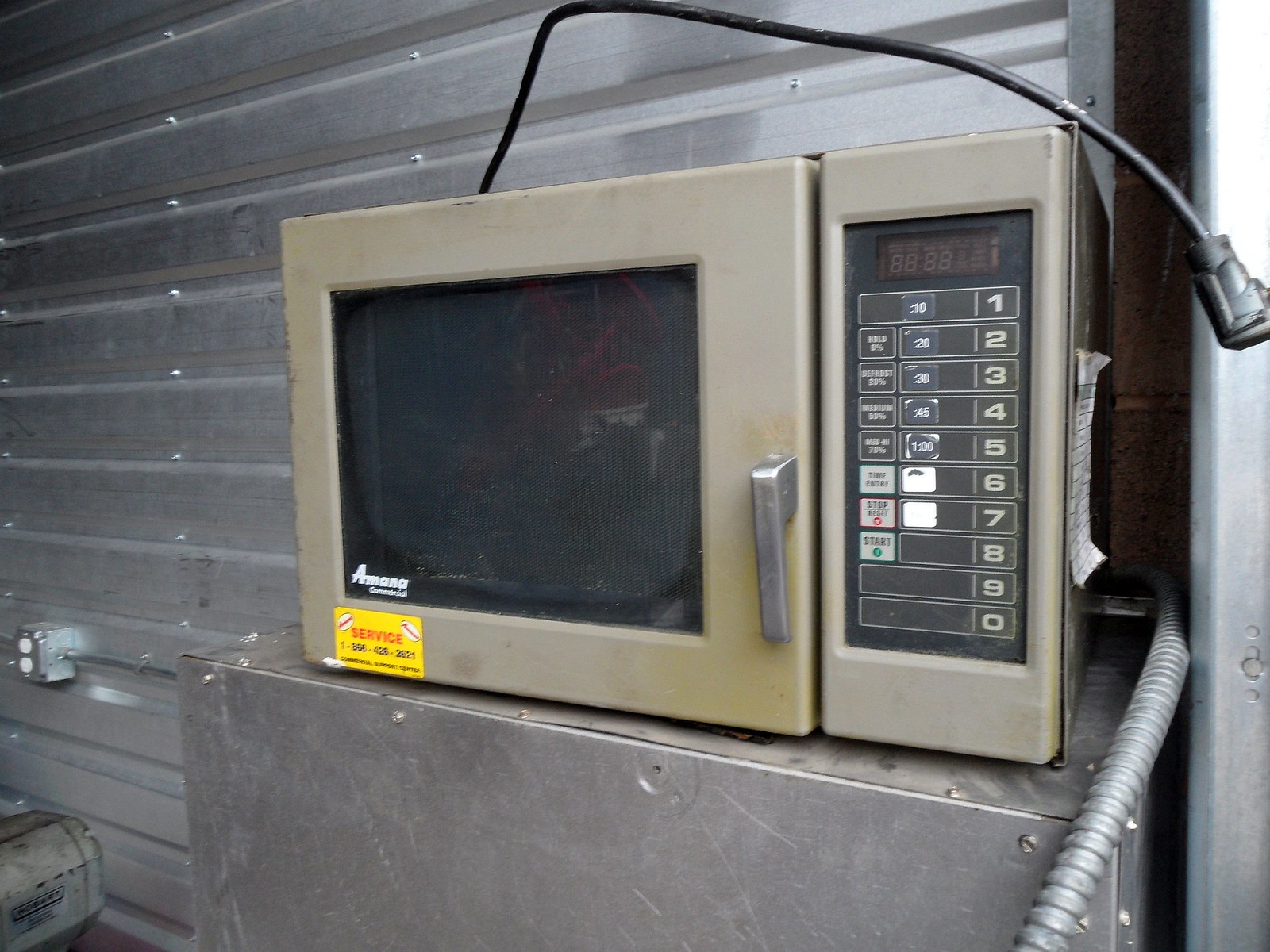This image showcases an old, visibly dirty microwave oven positioned in front of a corrugated silver metal garage door, resting on top of a silver metal platform. The microwave's surface exhibits light brown discoloration from accumulated dirt and age, particularly evident in areas frequently touched, such as the door and handle. The door, which swings outward, features a downward-bent chrome handle and a dark-tinted window. The bottom left corner of the door displays the brand name "Amana" above a yellow sticker labeled "service," with an illegible 1-800 number due to its small size. The right side of the microwave includes a control panel with rows of buttons numbered 0 through 9 in white. Additionally, some of the buttons have white squares, while others are empty. A power cord rests on the top right side of the microwave, beside a partially peeled-off label.